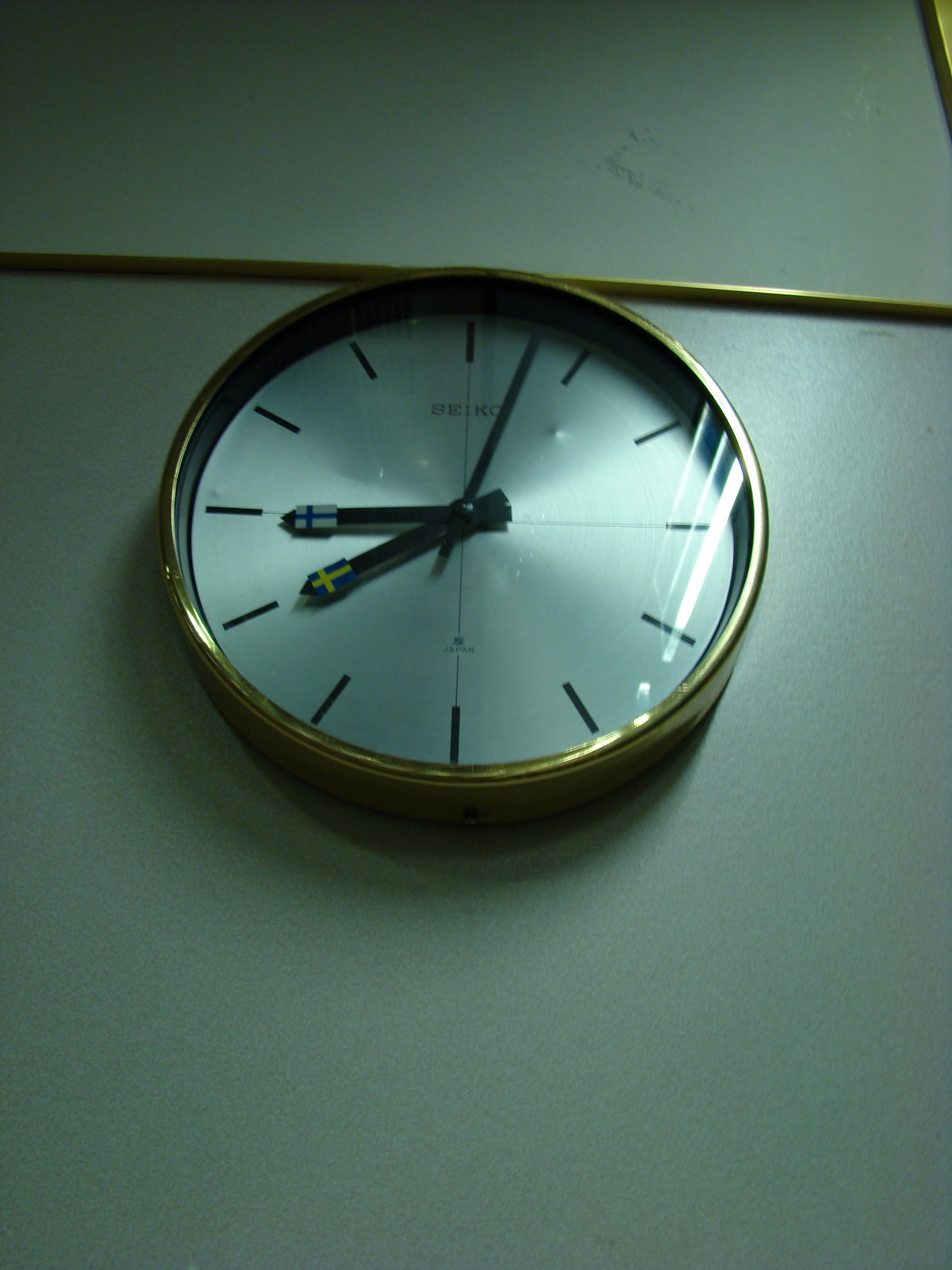The image depicts a centrally placed, round clock positioned on a subtly off-white wall. The wall has a darker sage hue with a blue undertone, and a fine gold line trim runs horizontally across the upper part of the image, forming a square border that frames the clock. The clock itself is encased in a gold frame and features a silver-toned face covered by a clear glass. The clock face is simple and minimalist, displaying only sleek black rectangular bars for hour markers instead of traditional numbered indices. Positioned at 8:40, the clock's black hands include hour and minute markers, each adorned at their tips with small flags: one flag is blue with a yellow cross, and the other is white with a blue cross. Additionally, a slim black second hand points between the 12 and 1 markers. Below the 12 o'clock position, the brand "Seiko" is printed in fine black letters, and near the 6 o'clock position, the word "Japan" is subtly inscribed. The clock hangs approximately at eye level, giving the impression of being viewed from a standing position.